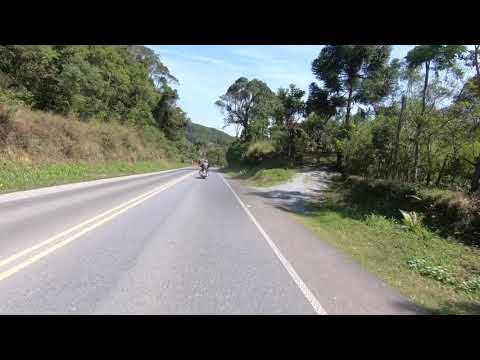The rectangular, horizontally oriented photo features an open road scene on a bright, clear day, bordered at the top and bottom by thin black lines. The road, a two-lane paved highway, stretches ahead with a double yellow line marking its center and a solid white line on its right-hand side. Nestled within the right lane, a motorcycle rider is visible in the distance, distinguished only by the silhouette and the rider's jacket. Surrounding this road are lush green embankments, tall trees, and dense greenery, with a dirt path splitting off to the right and ascending into the surrounding forest. The backdrop is a picturesque landscape of gently rolling hills under a brilliant blue sky, adorned with sporadic, wispy white clouds. The image contains a subtle blend of colors: the gray of the asphalt, the greens of the vegetation, and the blues and whites of the serene sky above.